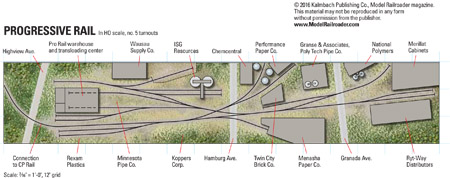This detailed, colored rail map vividly illustrates the intricate connections between rail lines and commercial facilities. The map prominently features black rail lines traversing the landscape, which is primarily depicted in green, denoting grassy areas, with brown hues around the rails. Roads are presented as gray strips, while buildings are illustrated as gray, black-outlined boxes. 

Detailed labeling is added for clarity, with small black text identifying specific locations. For instance, "Performance Paper Company" and "Granada Ave." are both marked with black text connected to their corresponding points via red lines. The title, "Progressive Rail," appears boldly in the upper left corner of the map. Although slightly out of focus, a copyright notice is visible in the upper right corner of the map. This comprehensive map offers a clear and insightful view of the rail network and associated commercial entities.